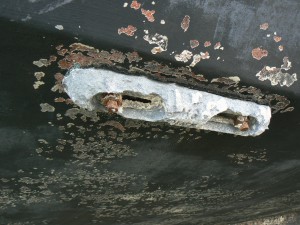The image depicts a corroded and rusted metal surface, possibly part of a boat or vehicle. The overall background is dark gray to black, heavily affected by rust and chipping paint. Central to the image is a white rectangular object, possibly an oblong piece of hardware, with two rusted screws or bolts securing it. Surrounding the white object, numerous slots or slits are visible. The entire scene is characterized by extensive pitting and peeling paint, with larger rust circles concentrated at the top and denser, smaller rust patches at the bottom right. The surface area appears compromised, with tan and black discoloration—potentially indicative of small organisms or extensive corrosion.